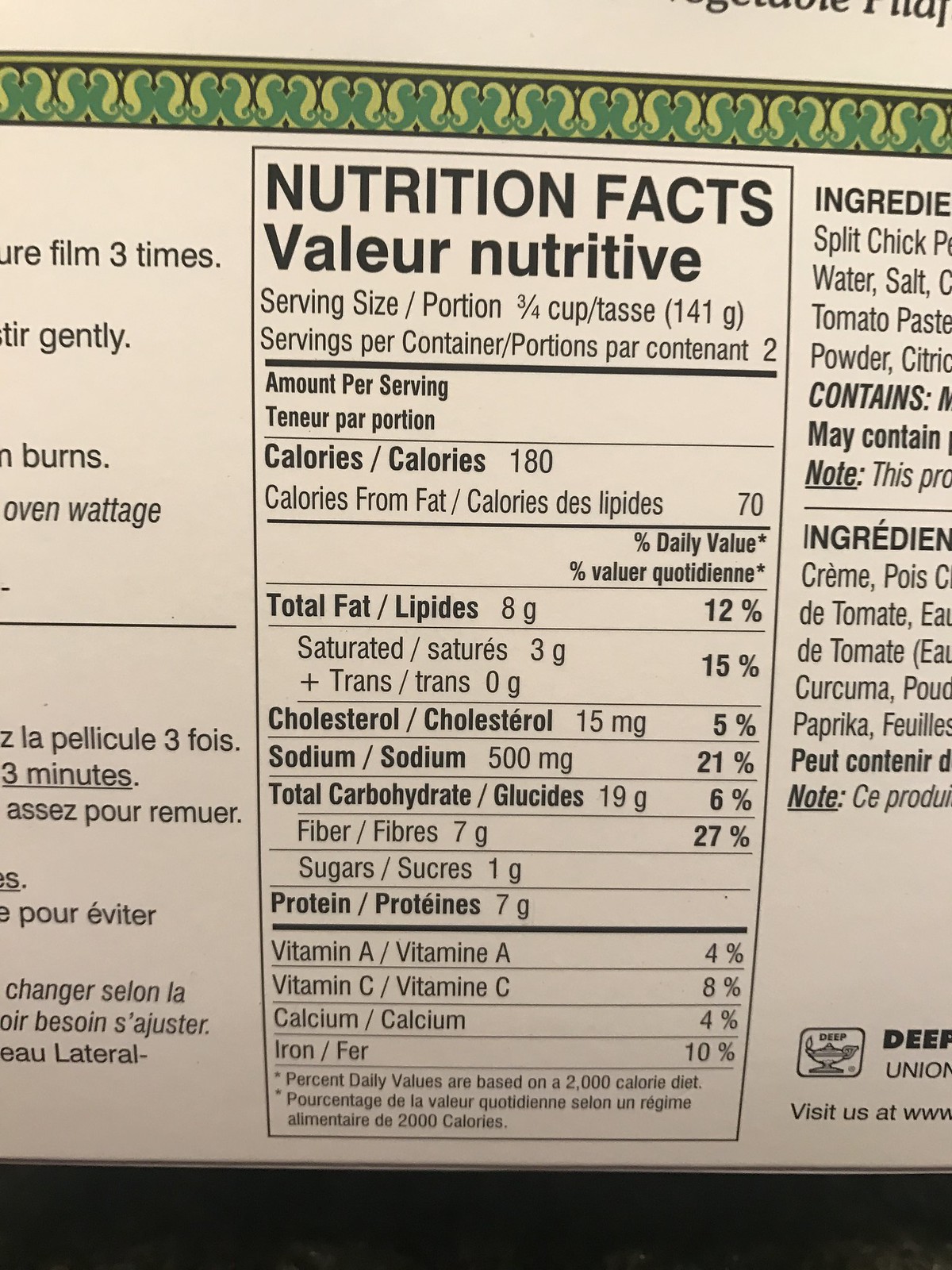The image depicts a detailed nutritional facts label, primarily in English, with some French translations. The label is printed on the back of standard food packaging. At the top, it prominently states "Nutrition Facts," followed by the French translation "Le Leur Nutritif." 

The serving size is specified as 3/4 of a cup, also noted in French as "Taster" (cup in English). Below this is a section titled "Amount Per Serving," detailing the caloric content and nutritional breakdown. It indicates that each serving contains 180 calories, with 70 of those calories coming from fat. This information is followed by a note that this is about 12% of the daily recommended intake.

Additional nutritional information is included, such as total carbohydrates and glucose levels, providing a comprehensive overview for consumers to understand the nutritional value of the food product.